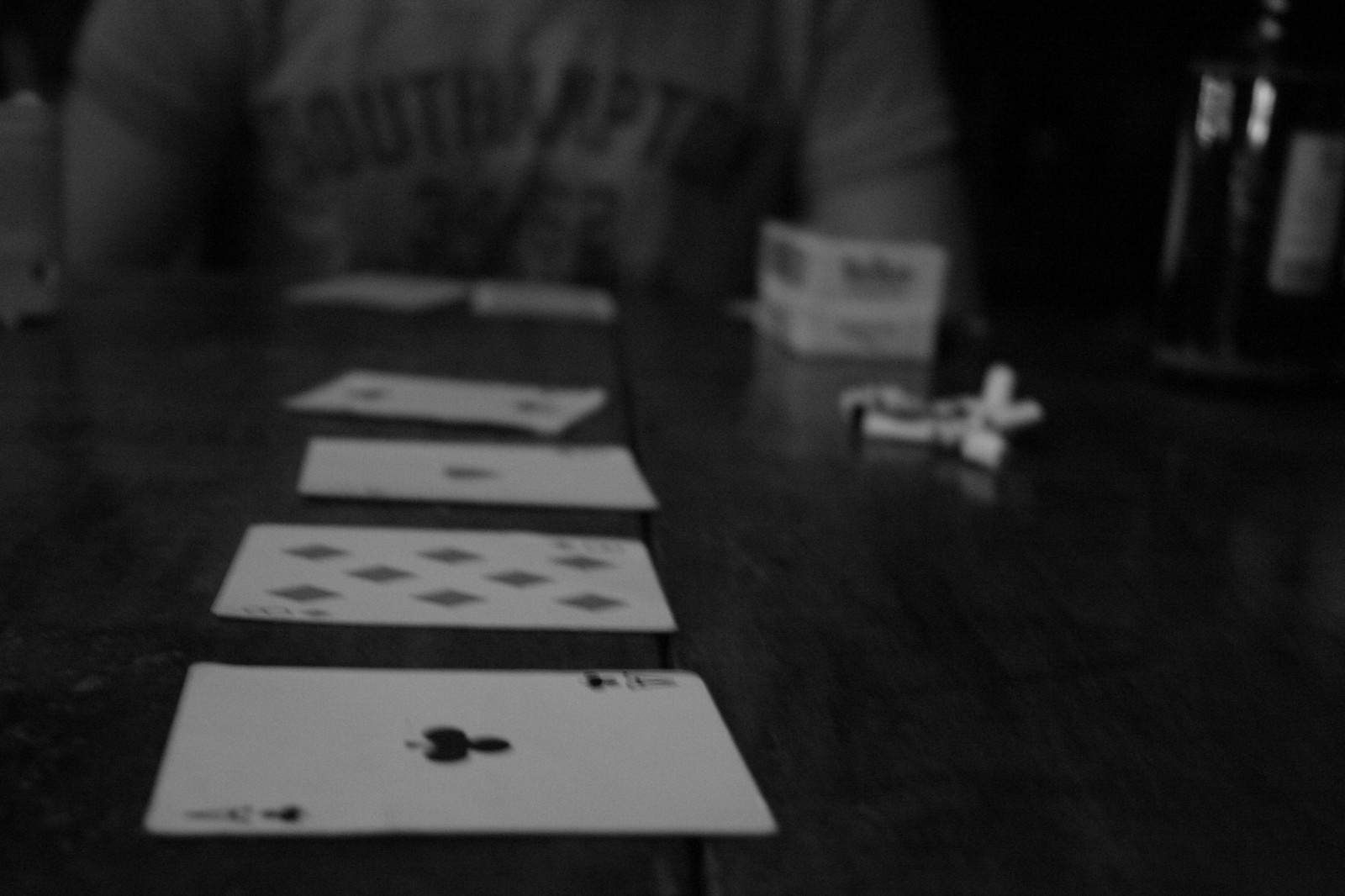In this evocative black-and-white photograph, a group of people are absorbed in a card game, with the primary focus on a wooden table, recognizable by a prominent seam running through its middle. Carefully arranged on the table are four playing cards: an ace of clubs, an eight of diamonds, an ace of hearts, and a two of clubs, which gradually blur into the background. Centrally placed among the cards rests an ashtray, heavily laden with spent cigarettes, suggesting an extended session of play and conversation. To the right, several bottles reflect the ambient light, hinting at leisurely indulgence. At the far end of the table sits a person wearing a short-sleeved T-shirt emblazoned with "South Raptor" and a possibly unclear number below. Before them lies an assortment of cards, contributing to the game's intensity. Adjacent to this individual are two indistinct boxes, potentially cigarette or card boxes, bearing some sort of logo. On the other side, a gray cylindrical object, which resembles a water bottle, completes the scene, adding a touch of everyday life to this moment of camaraderie and competition.